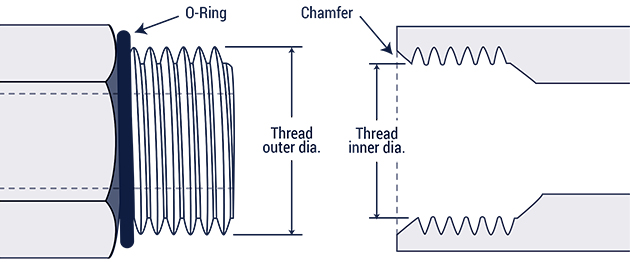This technical diagram on a white background illustrates the interaction between a screw and its corresponding threaded hole, both rendered in black outlines with gray shading in some areas. On the left side, a detailed drawing of a screw is annotated with "O-ring" pointing to a black band at the base of the screw threads. The screw's external grooves are labeled "Thread Outer DIA" with arrows indicating the diameter of the threads. On the right side, a matching diagram depicts the threaded cavity that receives the screw, labeled as "Chamfer" near the top right with an arrow pointing to the chamfered edge of the cavity. The interior measurement of the cavity's threads is marked "Thread Inner DIA," with arrows outlining this inner diameter. The center area where the threaded screw would be inserted remains white, representing the empty space. The diagram uses solid and dotted lines along with directional arrows to clarify the various components and measurements.